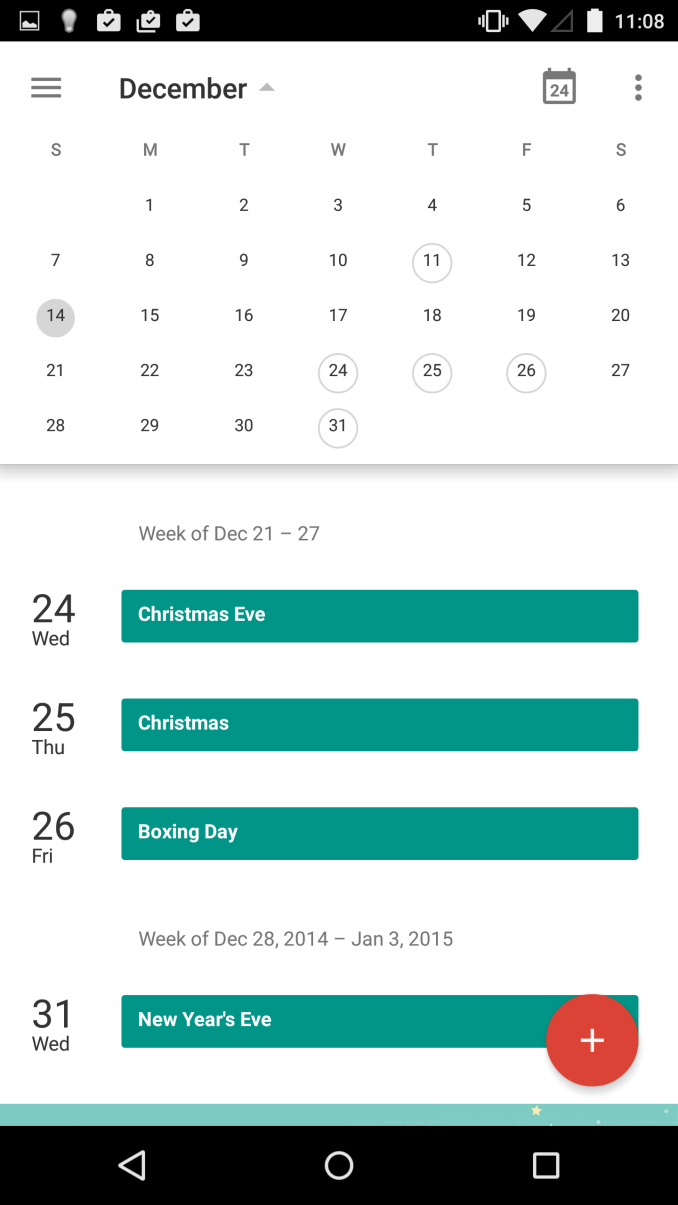This is a screenshot of a calendar app interface on a mobile phone. The interface features a dark header cluttered with icons on both the left and right sides. The main portion of the screen has a white background. 

At the top section, the calendar displays the month of December. On the left side of this section, three horizontal gray lines are visible. To the right of these lines, the text "December" is displayed prominently in bold black letters. Adjacent to this, a gray upward-pointing arrow is present. Further right, there is a calendar icon with the number 24 displayed on it, followed by three vertical gray dots.

Below this top section, the seven abbreviated days of the week (S, M, T, W, T, F, S) are listed horizontally. The calendar grid begins with "1" under M (Monday) and continues sequentially to "31" under W (Wednesday). Specific dates – the 11th, 24th, 25th, 26th, and 31st – are circled with thin gray lines, and the 14th is highlighted with a light gray circle.

Beneath the calendar, a faint shadow is visible, adding a subtle depth to the interface. Below this, a section labeled "Week of December 21-27" appears, featuring four horizontally highlighted teal blue lines with white text. The first line lists "24, Wednesday, Christmas Eve," the second line, "25th, Thursday, Christmas," the third line, "26th, Friday, Boxing Day," and then there is a header break indicating "Week of December 28, 2014, through January 3, 2015." The final line in this section lists "31, Wednesday, New Year's Eve."

At the bottom right corner of the screen, there is a red circle featuring a white plus sign, likely indicating an option to add a new event.